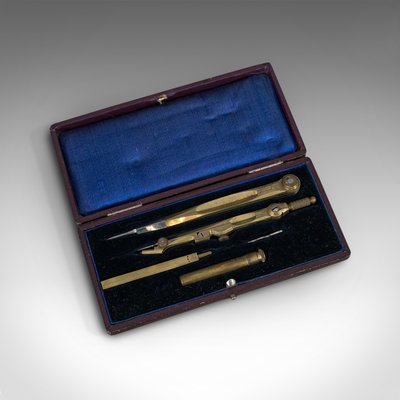The image depicts a small, rectangular carrying case, which is currently open and centrally positioned but slightly tilted to the left on a white and grayish background. The exterior of the case is purplish, with a blue padded lining on the inner side of the top lid. The interior bottom of the case is lined with black velvet-like material. Inside the case, four to five long, scalpel-like metal objects are neatly laid out. These instruments vary in color, displaying both brass and silver hues, with some having silver tips. There is also a golden or silver closure clip visible on the case. The objects appear to be precise tools, possibly related to music or another form of intricate work, but their exact purpose is unclear. The image has no associated text.